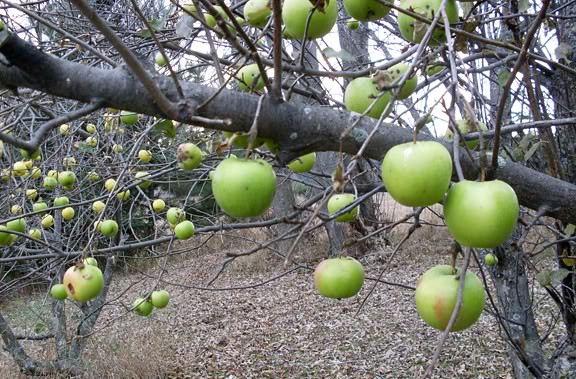This photo captures a detailed scene of an apple tree with several green apples, similar to Granny Smiths, hanging on its branches. A large, gray branch prominently crosses through the middle of the image, surrounded by numerous thinner branches that hold the green apples. Notably, the tree lacks leaves, suggesting a late fall or early winter timeframe, with dry brown leaves scattered uniformly across the mulch-like ground. Behind the apple-laden branches, there's a bright, light background that could be either the sky or another light source. Additional trees are visible in the background, which do not appear to be apple trees, hinting at a more forested area with a possible field beyond. It is also possible that the thick branch dominating the scene is from a different tree, and the apple tree is leaning onto it, supported further by a secondary apple tree visible in the bottom left part of the photo.